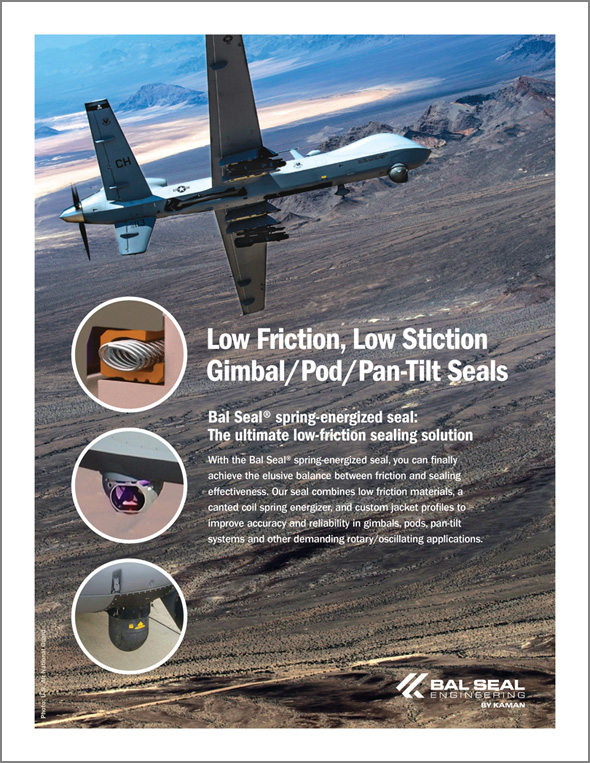This vertically oriented advertisement for BAL Seal Engineering showcases a small, blue military-style drone flying sideways over a rocky, desert landscape at either sunrise or sunset, with the view of foothill mountains in the background giving the scene a serene yet rugged ambiance. The image is bordered in white, and the photograph is realistic, capturing the detailed textures of the rocky environment. Central to the poster is bold white text promoting BAL Seal's advanced engineering solutions: "Low Friction, Low Stiction Gimbal/Pod/Pan Tilt Seals." Below this, in smaller white text, it elaborates, "BAL Seal Spring Energized Seal, the ultimate low friction sealing solution." Additional, albeit partially obscured, text describes how their custom jackets and canted coil spring energizers improve the accuracy and reliability of various demanding applications including gimbals, pods, and pan tilt systems. The bottom of the poster reads, "BAL Seal Engineering," and is possibly signed by an individual named Naman. On the left side, three circular, zoomed-in graphics display detailed images of the engineering components being advertised. The overall design suggests a high-tech, precision-engineered product aimed at improving performance in aerospace and similar industries.